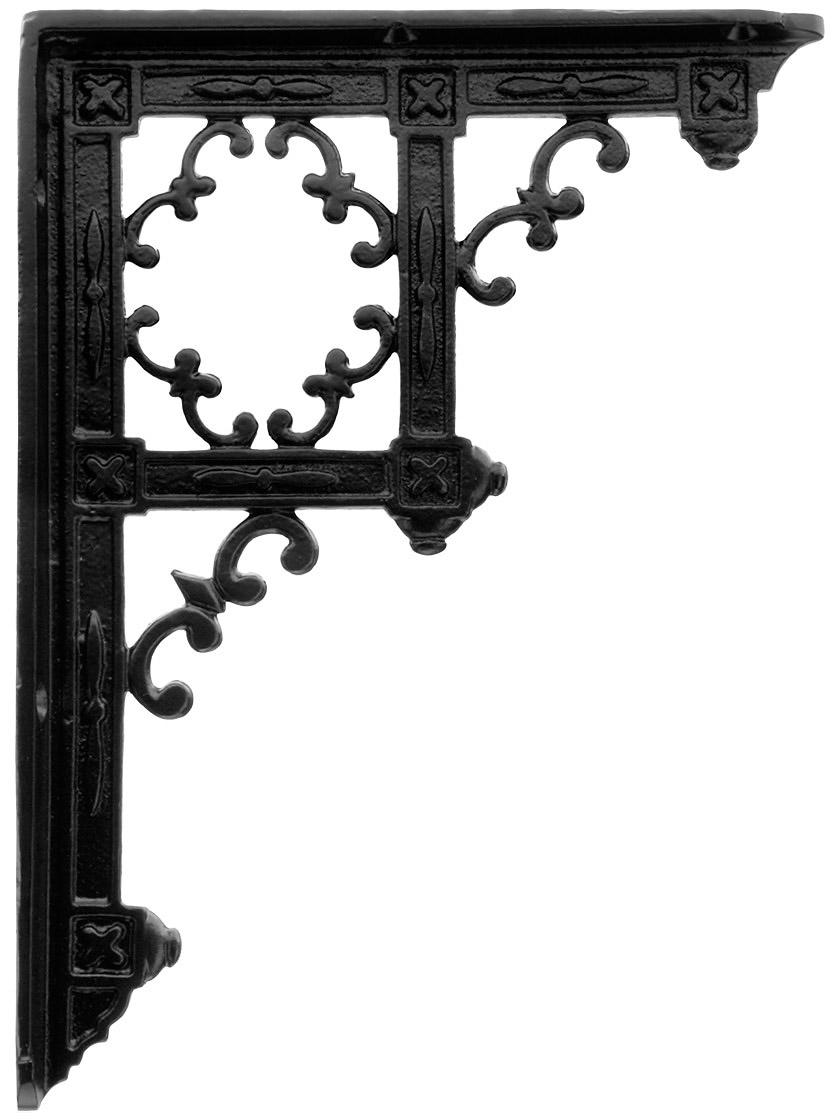The product displayed in the photograph is a black painted, right-angled bracket designed for commercial use, often seen in online shops, listings, or catalogs. This L-shaped bracket is made of metal, possibly cast iron, featuring decorative curved lines that give it a vine-like appearance. The bracket has multiple holes on the left and top sides to facilitate mounting, making it ideal for supporting shelves or other decorations against a wall. The intricate design includes various embellishments, such as X-shaped engravings and possibly clover or propeller-like symbols, adding to its aesthetic appeal. The photograph presents the product against a pure white background, creating a floating effect that highlights its detailed craftsmanship and practical utility.